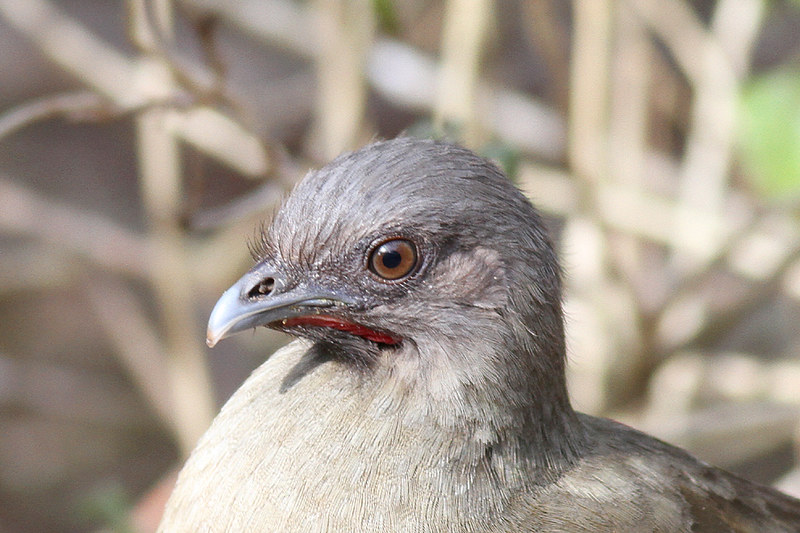This photograph features a detailed close-up of a plain chachalaca bird, captured from the chest up which provides an excellent view of its striking face. The bird stands upright, gazing to the left with focused brown eyes that have black pupils. Its head is predominantly gray, transitioning to beige on its body. It has a light gray beak with a noteworthy red streak stretching from beneath the beak to its cheek, giving it a distinct appearance. A subtle detail includes a bit of sand around its mouth and visibility into its nostril. In the out-of-focus background, beige twigs or branches are illuminated by sunny light, suggesting it may be in a tranquil, natural setting, possibly near ground level by a marsh or creek. The image is brightly lit, indicating it was taken during the daytime. The bird's wide-eyed expression adds an element of curiosity or surprise to its demeanor.